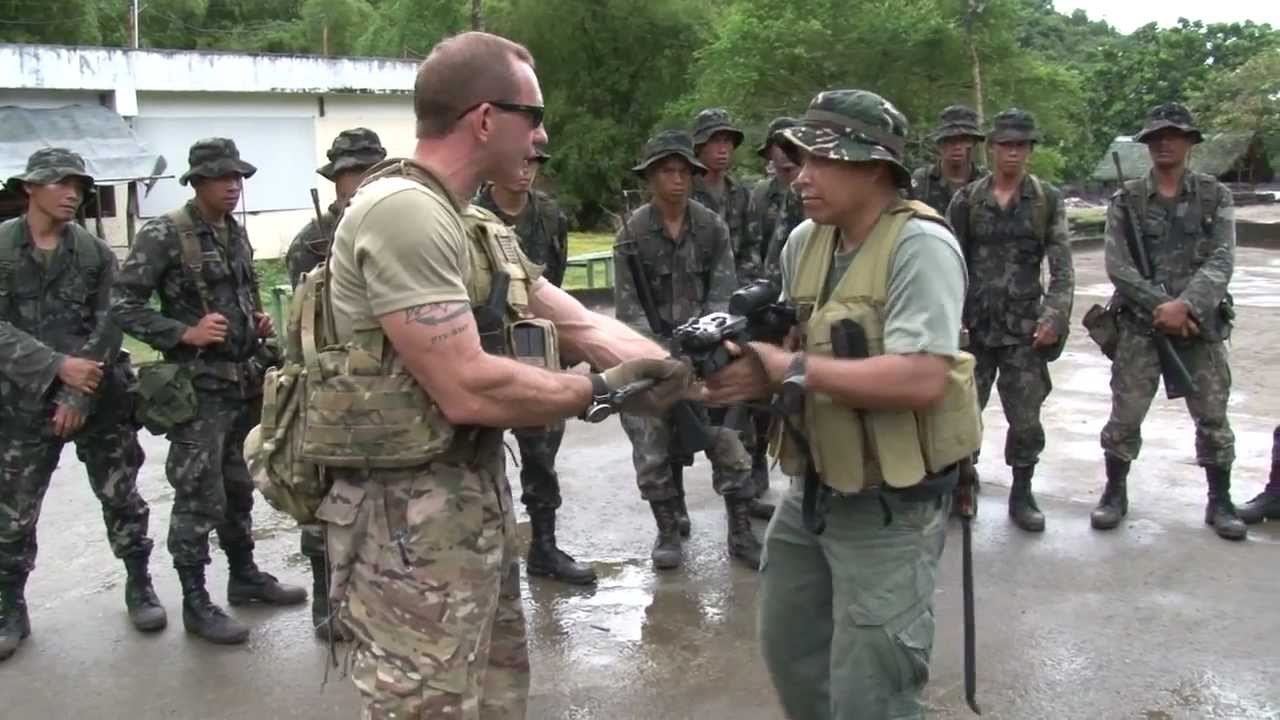This photograph captures a group of nearly a dozen soldiers lined up horizontally in the background, watching an interaction between two men in the foreground, set in an outdoor environment with green trees and a white building in the distance. The ground appears to be a solid surface, possibly concrete. The soldiers, all wearing camouflage uniforms and hats, exhibit a relaxed demeanor despite observing the activities upfront.

In the forefront, two men engage over a firearm. The man on the left, who appears Caucasian, is wearing a light short-sleeve green t-shirt, khaki pants, and dark sunglasses. He has a short haircut, a tattoo on his right arm, and is robustly built. He also carries a backpack and seems to be instructing or handing over the gun to the man on the right. The man on the right is donned in camouflage, with a khaki or camouflage green hat, and light green pants. The scene suggests a demonstration or training session rather than a conflict, evident from the composed posture of the bystanders.

The collective attire of the soldiers, including black boots and vests, underscores a coordinated military setting. The surrounding greenery and the white building frame an atmospheric backdrop that adds depth to the image.